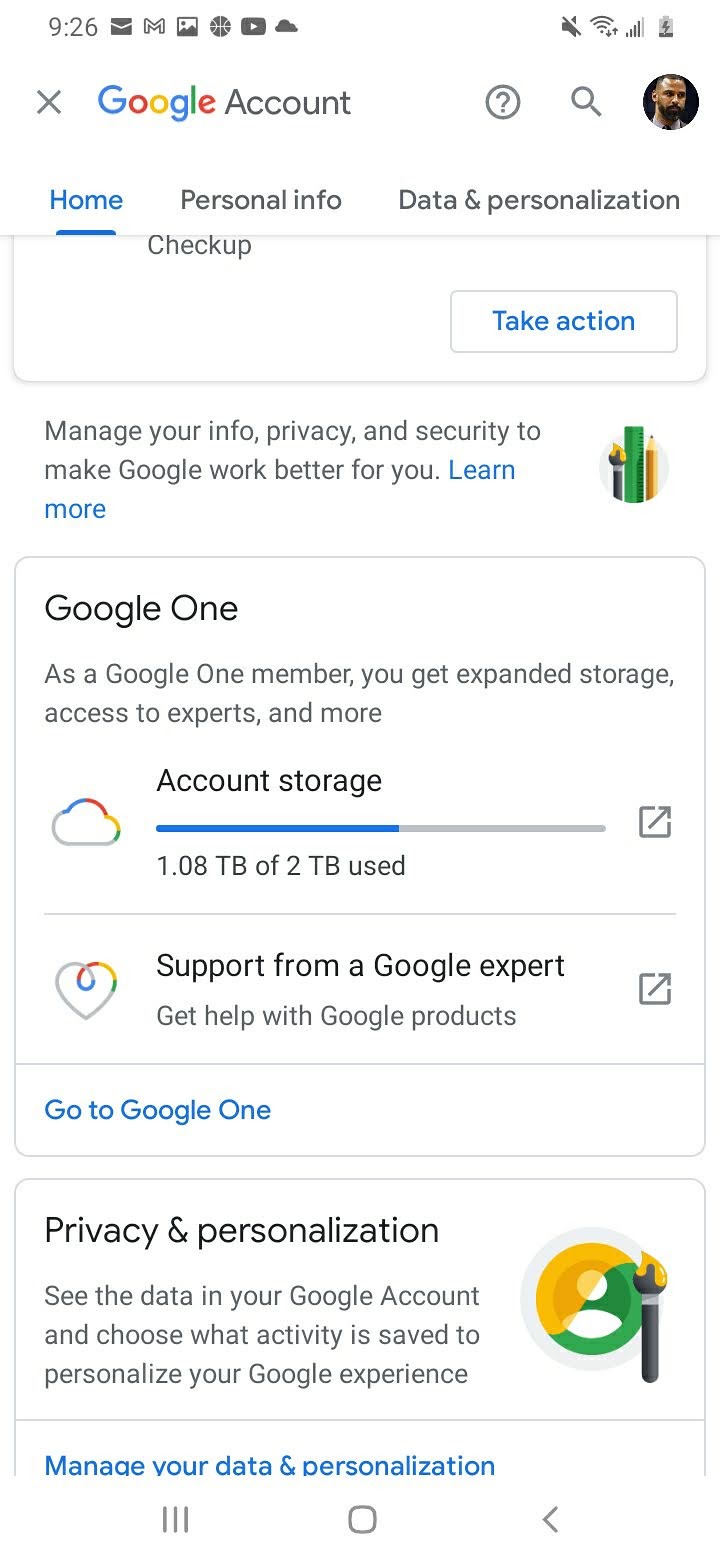This image is a detailed screenshot of a smartphone displaying the Google Account settings screen. The screenshot captures various elements typically found on a mobile device. At the very top, a standard status bar shows the time as 9:26, along with small icons indicating active apps, battery life, Wi-Fi strength, cellular signal, and silent mode.

Beneath the status bar, the screen is predominantly white with the Google Account interface prominently displayed. A circular profile picture signifies the user's account, with "Google Account" serving as the heading. The home setting is active, and other tabs labeled "Personal info" and "Data and personalization" are visible.

As the screen scrolls down, a section titled "Manage your info, privacy, and personalization" takes up the lower half to two-thirds of the image. Below this section, a gray border outlines the Google One account storage details, indicating that 1.08 terabytes out of 2 terabytes have been used. An option for support from a Google expert is also available with a clickable link labeled "Go to Google One."

At the very bottom of the screen, there's a "Privacy and personalization" section, followed by a link prompting the user to "Manage your data and personalization."